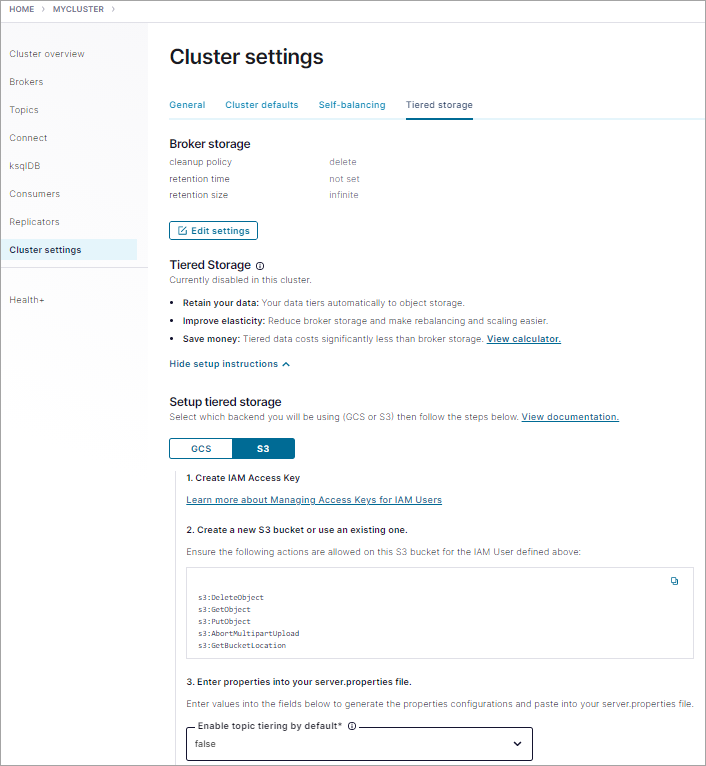A detailed caption for the provided image could be:

"This is a screenshot of the 'My Cluster' interface, specifically showcasing the 'Cluster Settings' tab. The screenshot reveals various cluster management options, including 'Broker Storage' and 'Tiered Storage,' with a section to set up tiered storage configurations. Small text under these headings likely provides detailed settings and options. The interface includes additional navigational tabs such as 'Cluster Overview,' 'Brokers,' 'Topics,' 'Connect,' 'KSQLDB,' 'Consumers,' 'Replicators,' and a 'Health' tab, indicating comprehensive management capabilities for data storage and server functionalities. It seems designed for administrators to monitor and configure the different aspects of data handling and storage in a clustered server environment."